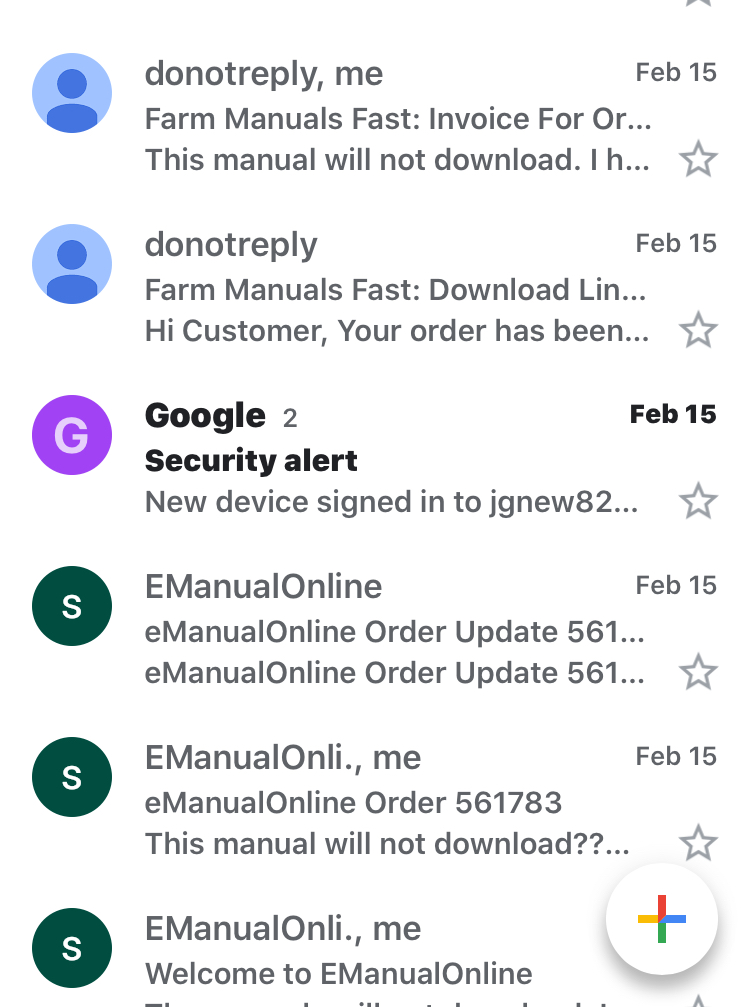The screenshot showcases an email inbox, likely from the Gmail app, given the bottom-right plus sign adorned in Google's signature colors of red, yellow, blue, and green. 

The inbox displays six emails, all dated February 15th. The first email is from "do not reply," associated with Farm Manuals Fast, featuring the subject "invoice for something" and mentioning that a manual did not download. 

The second email, also from "do not reply" at Farm Manuals Fast, addresses the customer with, "Hi customer, your order has been..." suggesting a continuation from a previous message or perhaps an order update.

The third email is a security alert from Google, notifying the account holder of a new device sign-in, which could indicate a new phone or gadget access.

The last three emails in the screenshot are from "emanualonline," though no specific details about these messages are provided.